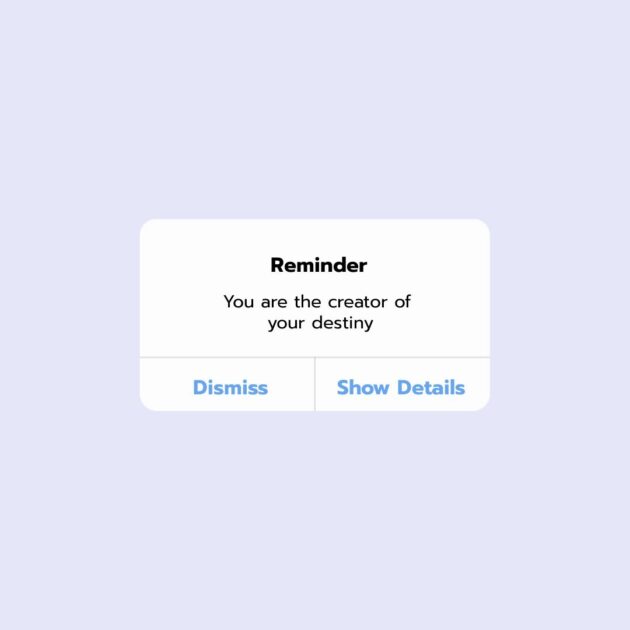This image is a closely-cropped screenshot of an unidentified digital interface, either a website, web application, or software application, showcasing a small notification dialog. Encased within a square-shaped box adorned in a pastel lilac purple background, the focus is a centered white rectangle. Dominating the top of this rectangle is the title "Reminder," rendered in bold black text. Below the bolded heading, a motivational message in smaller black text reads: "You are the creator of your destiny." Beneath this inspirational note, two actionable buttons are displayed: "Dismiss" and "Show Details," both presented in a bright blue bold text. The layout and color scheme of this notification dialog—featuring a harmonious blend of pastel lilac and white, accented with blue text for interactivity—provide a clean, modern aesthetic that could serve as an example for application design.